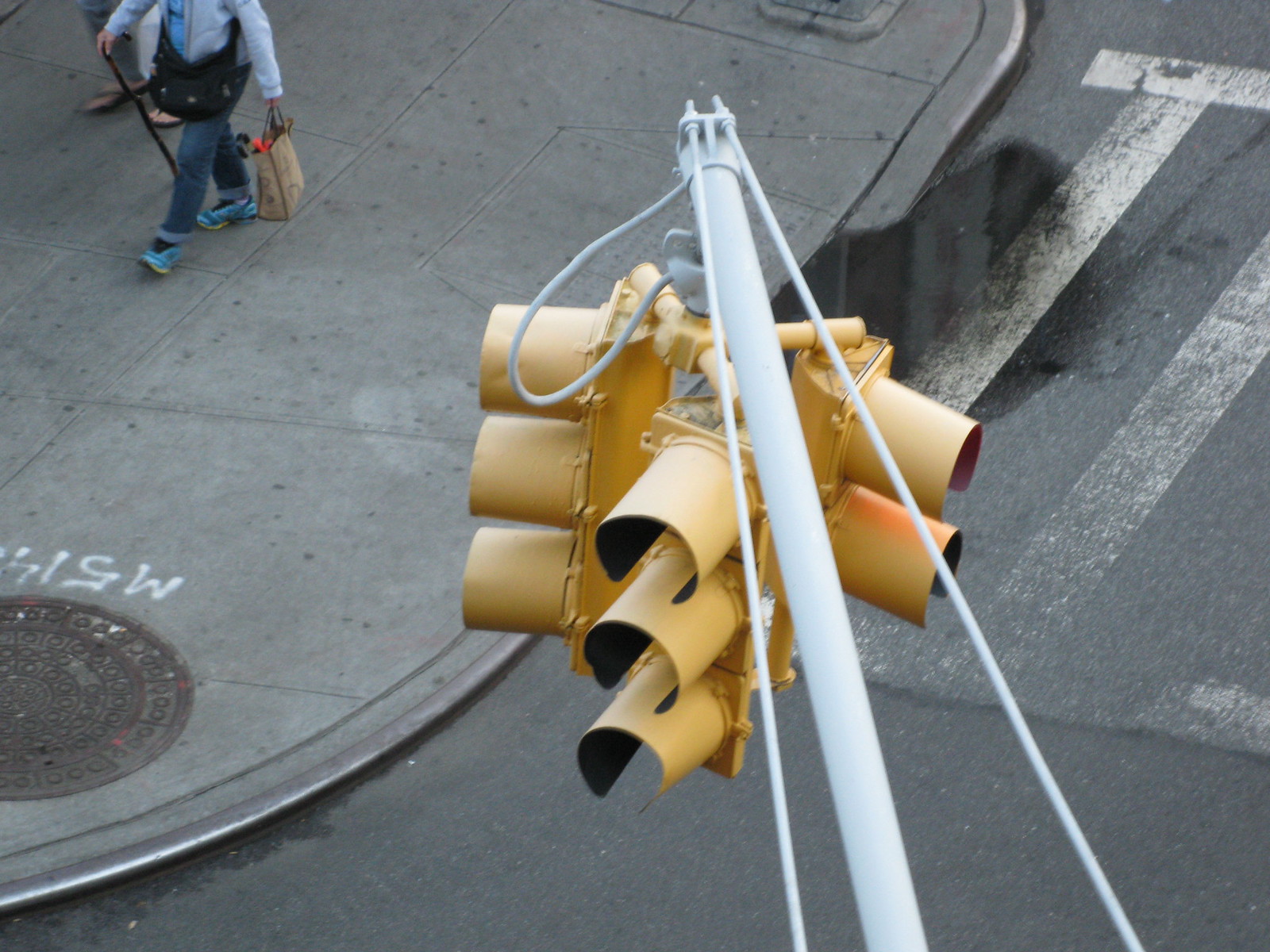A high-angle view captures a bustling urban scene, centered on a multi-directional traffic control signal. The traffic lights, housed in tan-yellow enclosures, extend from a prominent white pole, directing vehicles and pedestrians from three different directions. Below, a portion of the crosswalk is visible on the right-hand side, while on the left, a sidewalk hosts a solitary pedestrian. This individual, whose face remains unseen, is walking with a cane in their right hand and carrying a bag in their left, with another bag slung across their front. Water pools near the base of the sidewalk, hinting at the presence of a storm drain that facilitates drainage from the road below. The intricate details of this urban intersection paint a vivid picture of daily life and infrastructure at work.